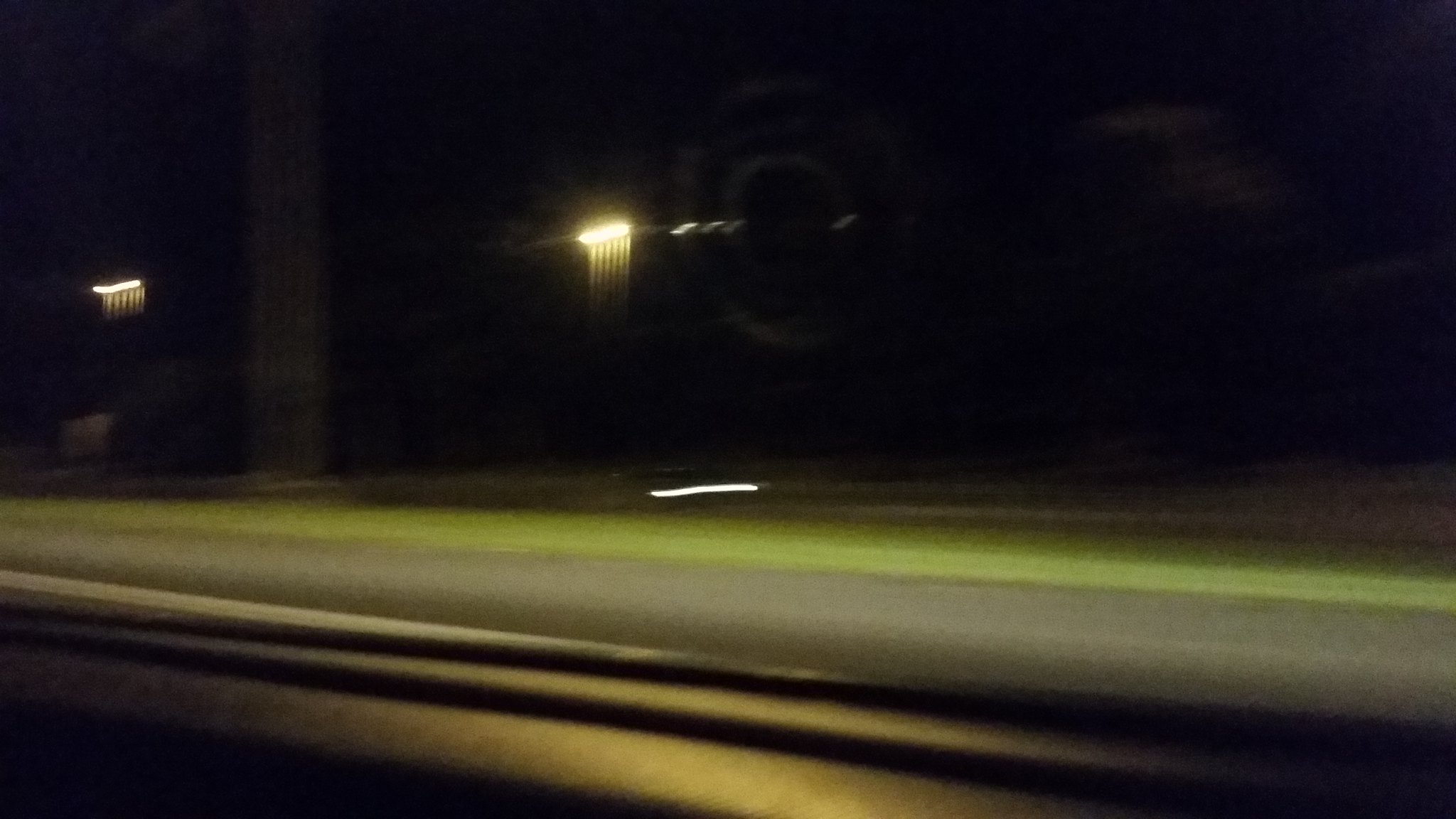A grainy and dark outdoor color photograph taken at night from a moving car. Entering from the left and extending horizontally across the lower half of the image is the side of the road, bordered by grass. The upper half of the photograph is predominantly black, with few discernible details. Just left of center in the upper half, there is a blurred, illuminated streak from an overhead streetlight, paralleled by a similar horizontal light line closer to the left edge. Near the center, slightly left of center, another horizontal light streak approximately a meter long is visible. The image lacks any text or print and doesn't show any reflection of the car window, reinforcing the candid, in-motion capture of the scene.